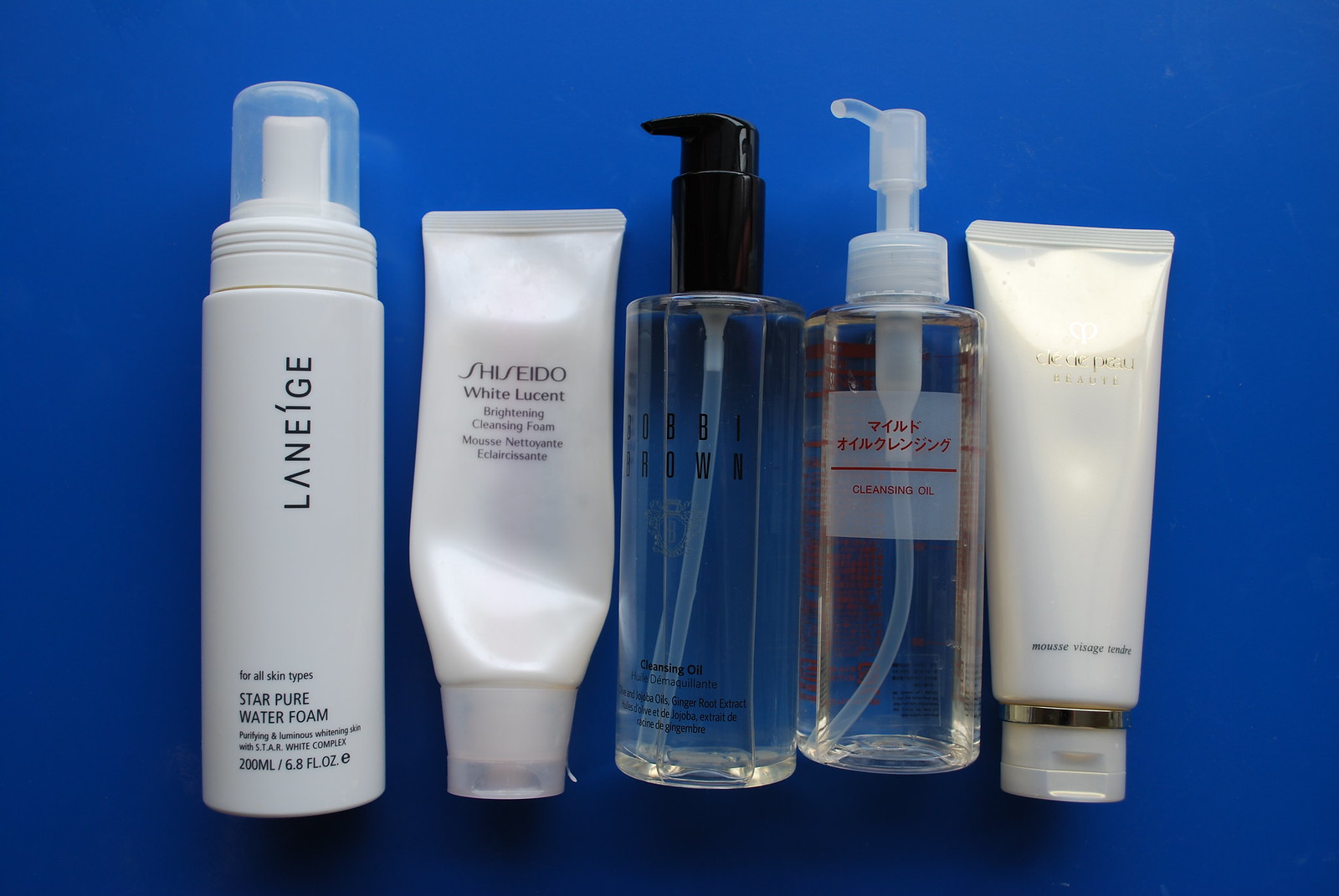In this vibrant blue background sits an array of five diverse beauty products, meticulously arranged for a close-up view. The first item on the left is a sleek, white bottle of Laneige's 'Star Pure Water Foam,' boasting a capacity of 6.8 ounces. Topped with a cap, this product is designed to dispense a foaming cleanser suitable for all skin types.

Next to it stands a rectangular tube that appears pocket-sized, hinting at a multipurpose function like a mini sunscreen or hand cream. It is a partly-used tube of Shiseido's 'White Lucent Brightening Cleansing Foam,' featuring text in English and another language, possibly French. The white tube indents at the bottom, suggesting it's a sample size.

Centrally positioned is a bottle of Bobbi Brown's 'Soothing Cleansing Oil,' distinguished by its clear liquid content and a black pump top. Adorned with text in multiple languages, it highlights ingredients like jojoba oil and ginger root extract.

To its right is another clear pump bottle, this time with a white pump cap. The bottle contains a lightly tinted brown cleansing oil, with red lettering and a red line accent. The text appears to be in a Japanese script, adding an exotic touch to the collection.

The final product mirrors the second in size and shape, resembling a tube of hand cream. This elegant, ivory white tube is branded 'Clé de Peau Beauté,' featuring a heart-shaped logo divided by a line in the middle. The product name is accented with gold lettering and a sophisticated gold ring near the cap, giving it a touch of luxury. Each item in this ensemble offers a unique contribution to a comprehensive skincare routine.